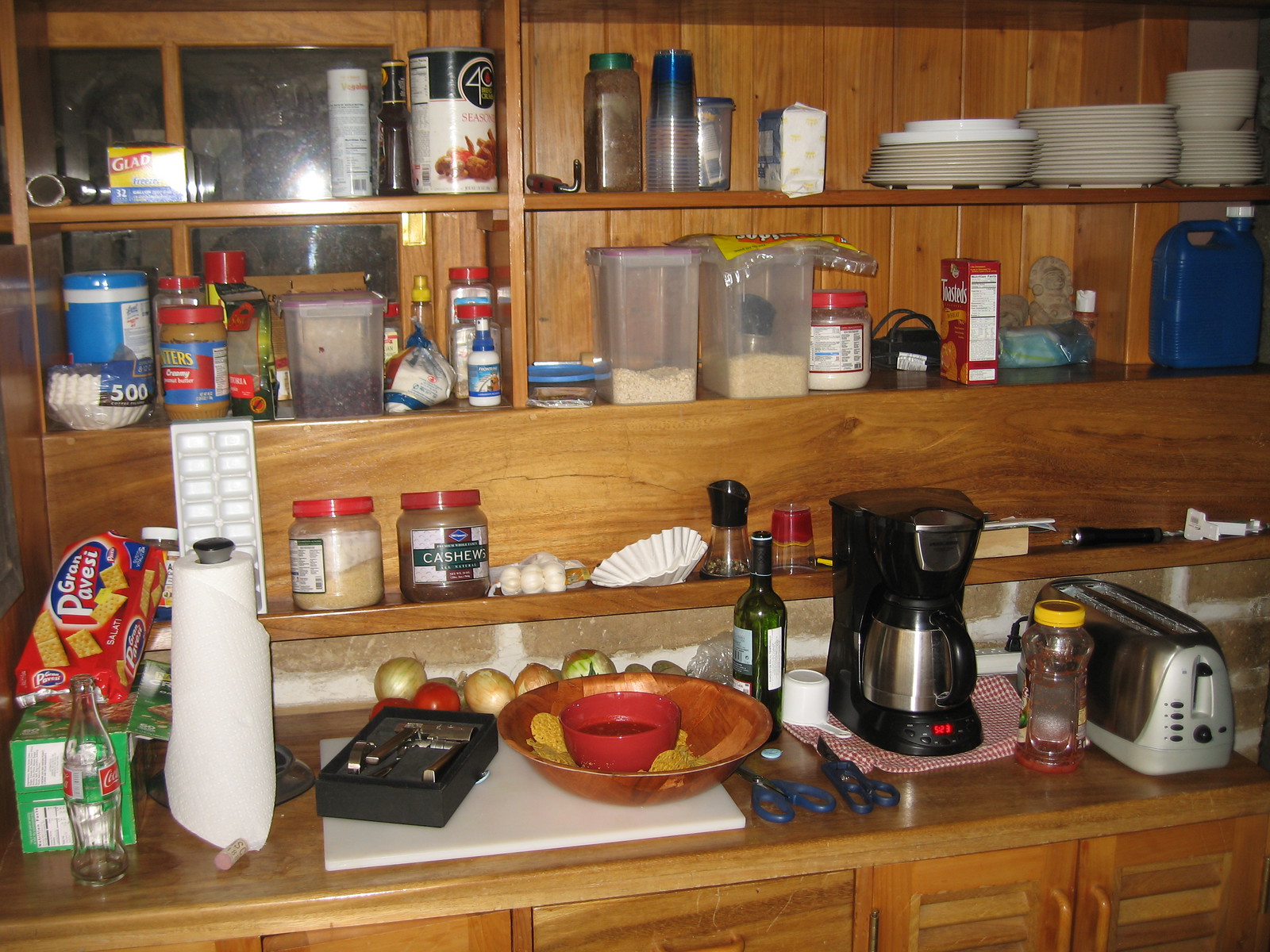The color photograph showcases a cozy kitchen corner, featuring an entire wall of honey-brown wooden elements including the counter, shelves, cabinets, and the wall itself, accentuated by visible knots and grains in the wood. The countertop is a bustling workspace, starting on the right with a jar capped in yellow containing a red substance at its base. Adjacent to this, a coffee maker rests on a red and white checkered cloth. Blue-handled scissors are placed next to a white upside-down measuring cup, while a green bottle, possibly a wine bottle, stands with its label turned away from the lens. A large, wooden strip-patterned bowl holds a smaller red bowl filled with tortilla chips. Further along, a black box with its lid removed displays an unspecified piece of equipment. 

Behind this setup, a roll of white paper towels is flanked by a scattered wine cork, an empty Coke bottle, and a green box of food. Subtle details like onions in the background contribute to the lived-in feel. Floating above, a shelf holds a white coffee filter, garlic heads, a plastic jar of cashews, and a white ice tray propped vertically. Ascending to the next shelf, one encounters a package of coffee filters, a jar of peanut butter, and several plastic containers filled with food. A jar with a red cap containing a white substance is also noticeable. The very top shelf stores a variety of kitchen essentials including saucers, dishes, bowls, plates, plastic cups stacked together, and a box of Glad freezer bags.

On the left-hand side of the photograph, a four-paned window peeks into the outside darkness, adding a touch of ambiance and concluding the holistic view of this inviting kitchen scene.